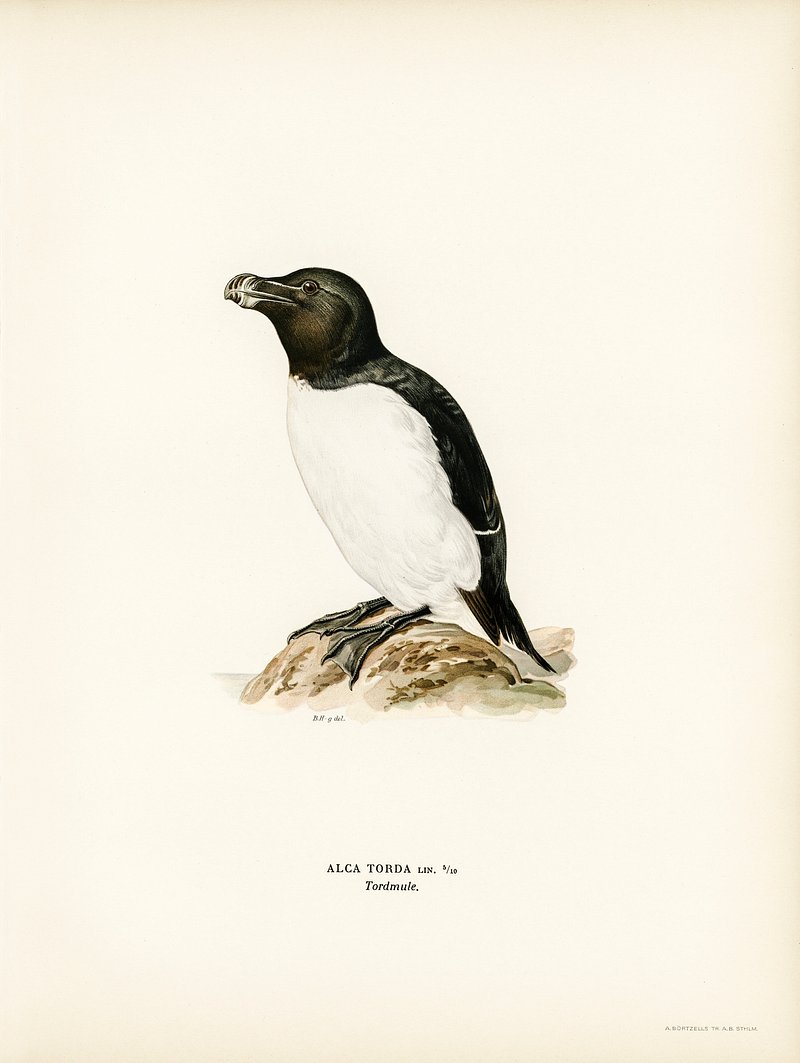This highly detailed drawing depicts a seabird that strikingly resembles a penguin. The bird, identified in the inscriptions beneath the image as "Alca torday" or "tort mule," is perched upon a brown rock that suggests a seashore setting. With a combination of black and white plumage, it features a white underbelly that starkly contrasts its dark head, back, and tail. The bird's webbed feet are black and complement its striking black or dark brown beak, which culminates in a blunted, somewhat whitish tip—a shape reminiscent of a cross between a pointed beak and a duck bill. The bird's rounded head hosts a small, dark eye, and its overall appearance evokes the style of classic illustrations, similar to those of Audubon, though not conclusively confirmed as such. The image is noted for its clarity and detailed artistry, making it a captivating portrayal of this seabird. Additional text in the bottom right corner, difficult to read, perhaps contains more descriptive or classificatory information.